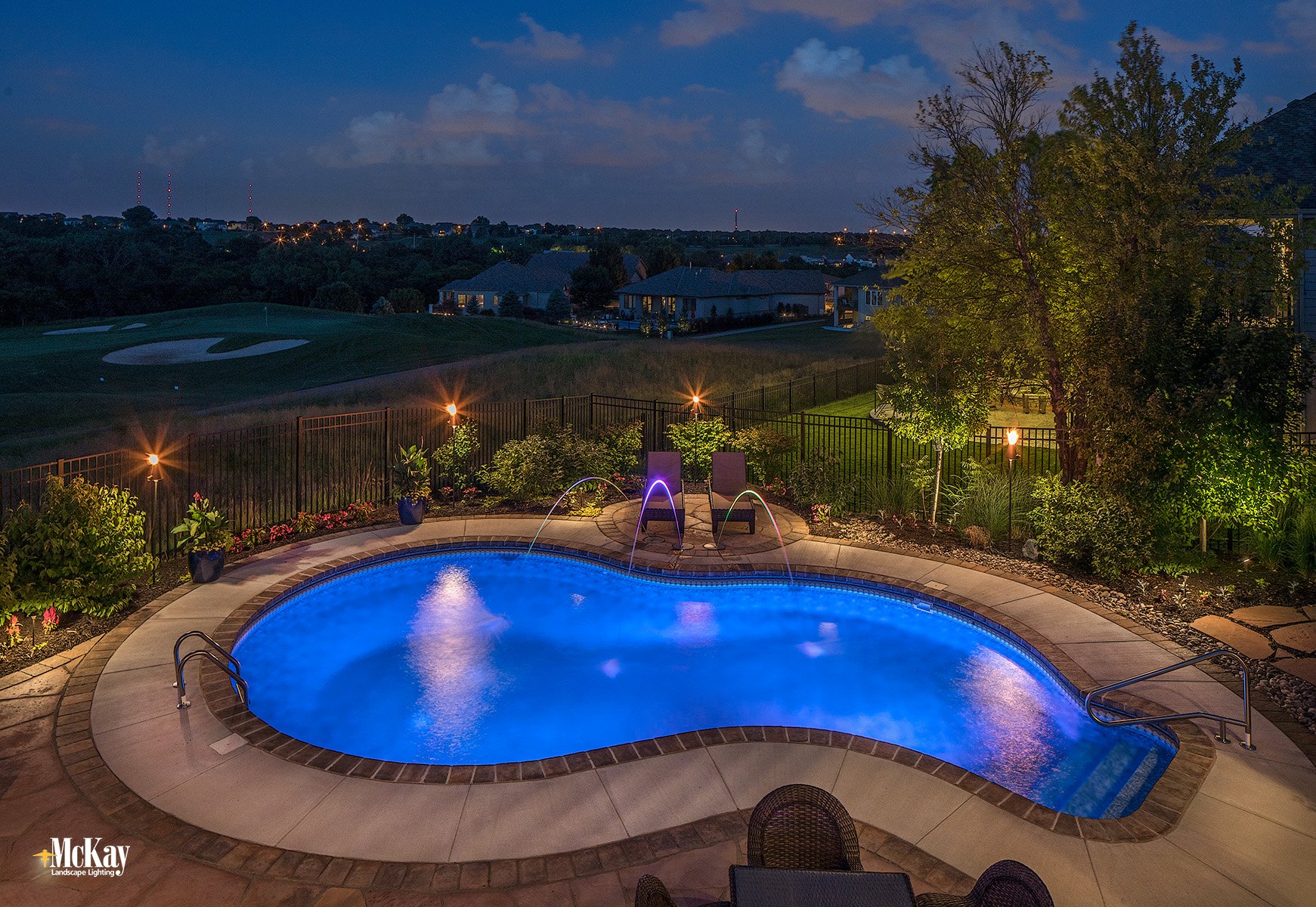This photograph captures a beautifully landscaped backyard setting, taken towards evening with a darker sky framed by a few lingering clouds. In the foreground, a prominently featured bright blue in-ground swimming pool curved in a peanut-like shape is lit from within, creating a warm, inviting glow. The pool has three water fountains gracefully arcing into it, and metal steps with a railing leading up to a marble or tile deck area.

Surrounding the pool, there is meticulous landscaping comprising decorative stones, vibrant shrubs, potted plants with flowers, and one notable tree. A black wrought iron fence encloses the area, complementing the serene environment. To the right of the pool, a brown table with chairs offers a seating area on the paver-lined patio, while two brownish chairs provide additional seating.

In the background, the scene stretches out to reveal a neighborhood characterized by scattered homes with illuminated windows, hinting at the evening setting. Beyond the homes, a golf course is visible with sand traps shaped like U's, enhancing the idyllic countryside feel. The presence of "McKay Landscape Lighting" text in the bottom left corner suggests professional lighting design, further accentuating the stylish and warm ambiance of this inviting outdoor space.